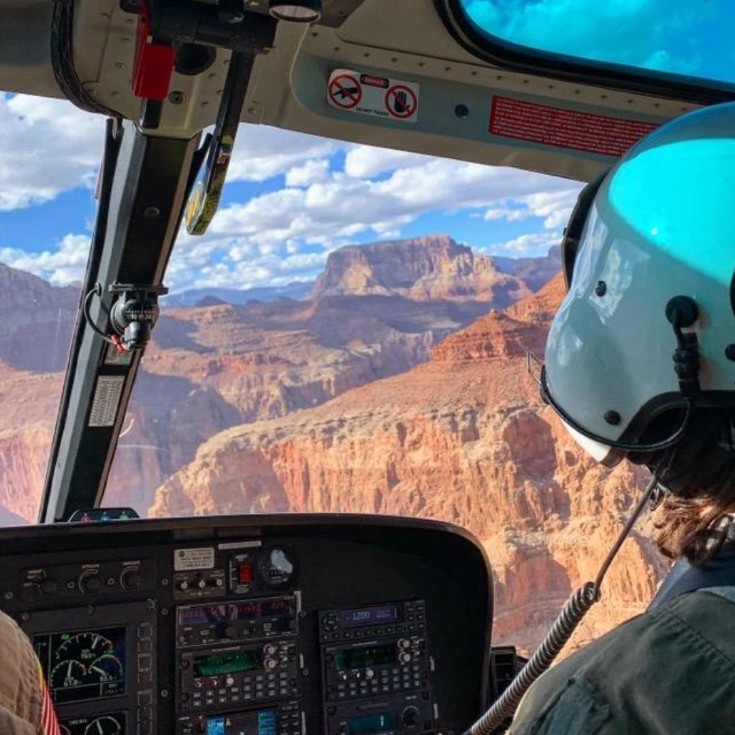This close-up photograph, taken from the back seat of a helicopter flying over the Grand Canyon, offers a striking view through the large front windshield. The scene outside showcases the Grand Canyon in all its majestic beauty, with rugged mountains, canyons, mesas, and plateaus bathed in the oranges and creams of the desert landscape. The blue sky above is adorned with broken, fluffy white clouds, casting shadows on the canyon rocks below.

Inside the helicopter, you can see part of the pilot’s right shoulder, adorned with a United States patch on desert camo clothing, and he is wearing a white helmet connected to the communications system via a curly cord. To the left, the co-pilot, in a green jacket and an aqua blue helmet, also has a cord running from the helmet to the dashboard. The intricate control panel, black with an array of whitish buttons and dials, is visible along with some skylights above the metal framework and a compass. The photograph captures both the technical interior of the helicopter and the breathtaking exterior vista, creating a vivid and detailed portrayal of the flight over the dramatic canyon landscape.